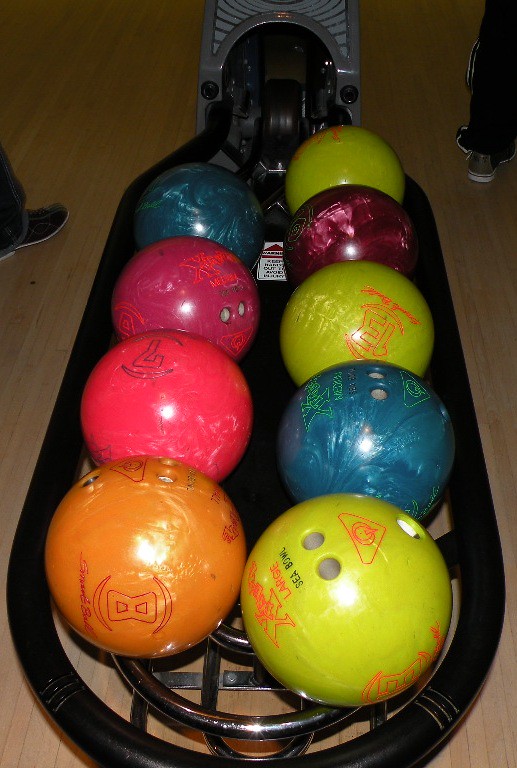This image depicts an indoor scene at a bowling alley, focusing on a close-up of the ball return mechanism. Flanked by sections of polished hardwood floor, the foreground is dominated by a horseshoe-shaped rack filled with nine colorful bowling balls. On the left side, a person's right leg clad in jeans and brownish-colored bowling shoes is visible, while on the right, another individual stands with their left leg in a track suit, also wearing bowling shoes. The ball return machine features a rubber piece that transports the balls back after they've knocked down pins, and in it, you find an array of bowling balls organized in two rows. From left to right, the balls are arranged in the following colors: three vibrant yellow balls (one labeled "large" and "seaball"), a sparkly blue ball, two magenta balls (with one appearing hotter pink than the other), a light orange ball, a deep reddish-pink ball, and another blue sparkly ball.